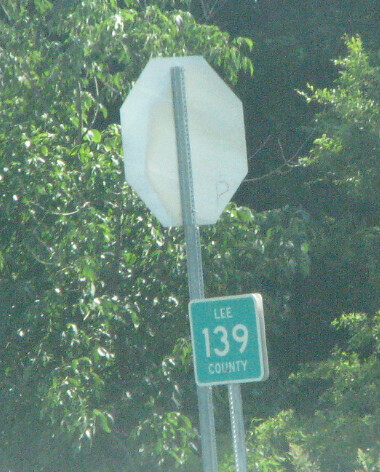The image depicts an outdoor scene with two distinct signs mounted on a single silver or gray pole. The top sign is an octagonal shape, showcasing a white back, typically indicative of a stop sign viewed from behind. Below it, a smaller, square-shaped sign is visible. This sign reads "Lee, 139 County" in white text. The backdrop is lush and verdant, filled with an abundance of green plants or leaves, enhancing the natural setting of the image.